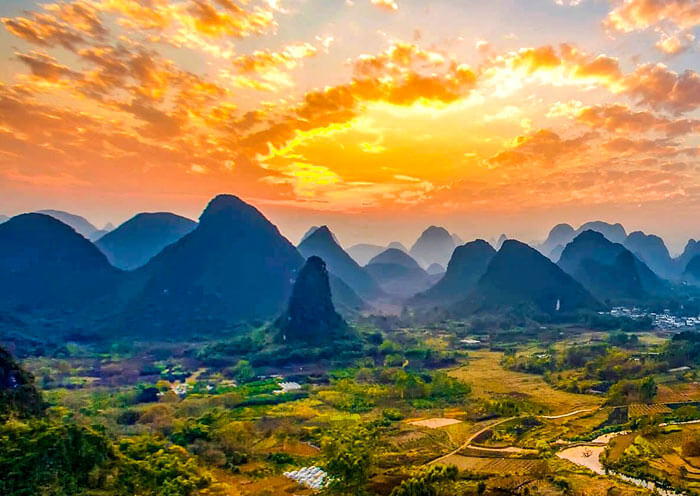The image depicts a breathtaking landscape at sunset, showcasing a sky painted with vibrant hues of bluish-pink, orange, and yellow. The majestic mountain range in the background transitions from the bright summit to darker tones as it descends. Numerous steep hills stretch out into the distance, layered with a fog that adds depth. In the foreground, lush greenery, dirt paths, and clusters of bushes and trees are visible. On the right side, a small village nestles among the terrain, marked by houses, fields of crops, dried pasture areas, and several roads. The bottom right corner features a winding river, while near the village, a parking lot full of cars can be seen. Overall, the scene captures the serene beauty of nature merging with small human settlements under a vividly colorful sunset sky.